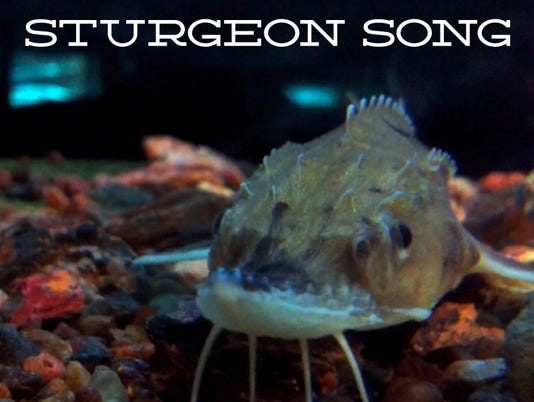The image, titled "Sturgeon's Song", features a detailed close-up of a sturgeon fish in an aquarium setting. The fish has a distinctive greenish-brown tone with a medium brown overlaid hue and visible scales. Its prominent features include black eyes, sharp white pointy teeth, and four white whisker-like appendages stemming from its chin. The sturgeon is surrounded by a colorful bed of rocks in shades of red, blue, clear, orange, light brown, and dark brown, indicating its low swimming position near the aquarium floor. The background appears dark with hints of a window's reflection, adding depth to the aquatic scene. The title "Sturgeon's Song" is displayed in white font at the top of the image, emphasizing the fish's identity and the overall serene yet mysterious ambiance created by the blue lighting within the tank.